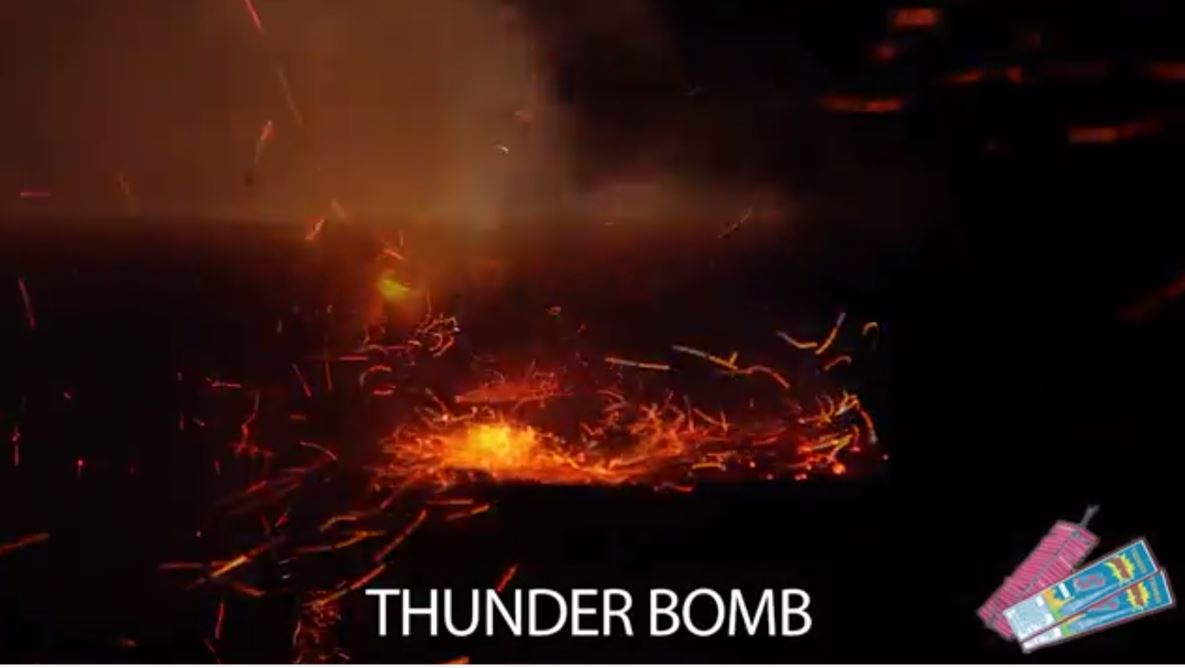The image is an advertisement for a firework named "Thunderbomb." Dominating the bottom right-hand corner are several pink, cylindrical sticks resembling hot dogs, bound together with a gray rope, representing the exterior of the firework. Encasing these sticks is blue packaging with textual details too small to discern, apart from the prominent white lettering of the firework's name: "Thunderbomb." The ad also features a dynamic visual of a recent explosion, presumably caused by the Thunderbomb, with a smoldering hole in the ground surrounded by vibrant red sparks and flames. This striking scene highlights the firework's powerful impact, capturing the viewer's attention with its fiery aftermath.